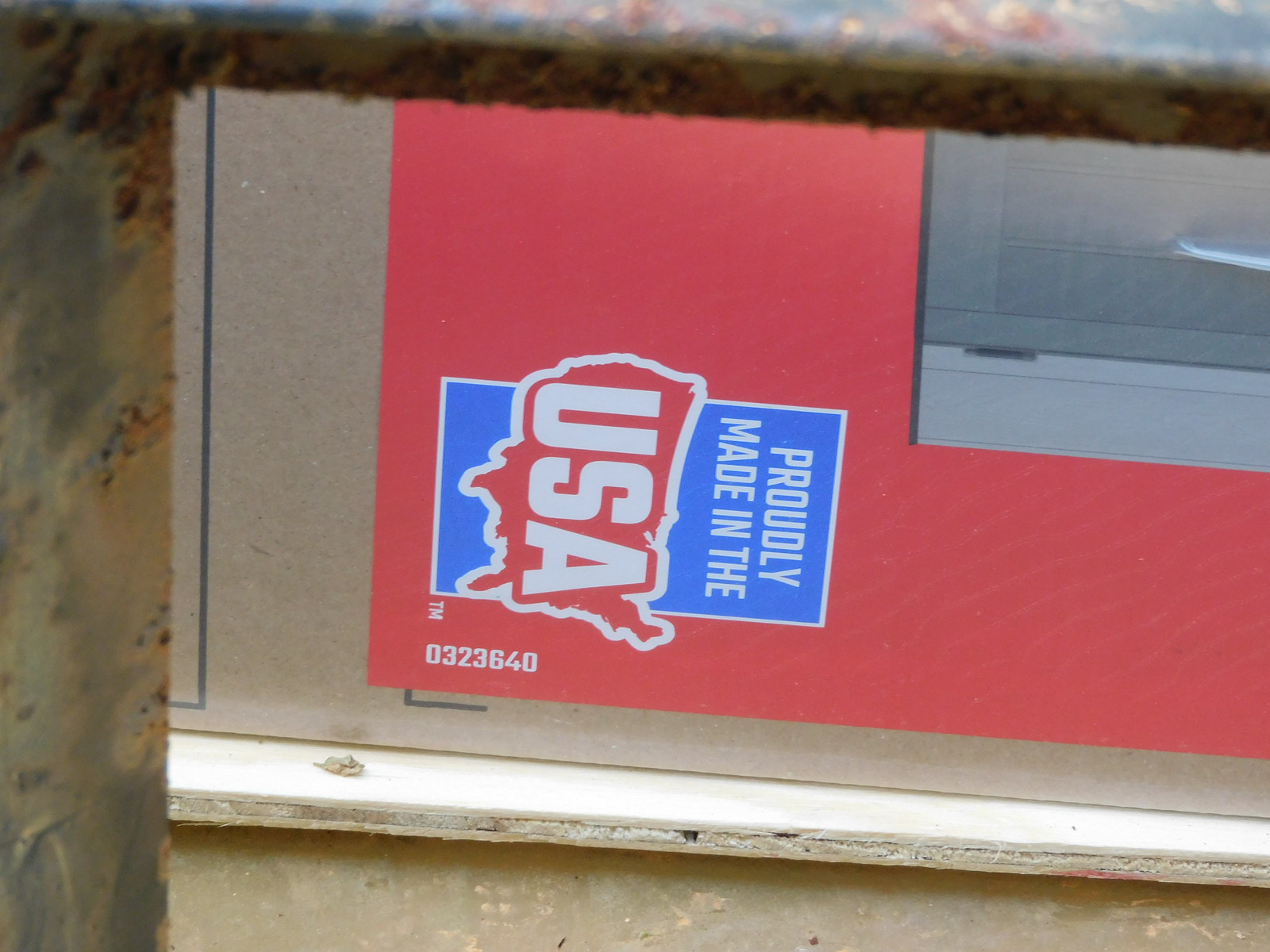The image is a wide, close-up photograph of a product's label on what looks to be a cardboard box. The box, tilted on its side, features a red background with a blue, vertical rectangle housing white text. Dominating the design is a red silhouette of the United States, with the words "Proudly Made in the USA" written in white across the map. Below this, a series of numbers resembling a serial or model number is present. The label sits amidst a rustic setting, possibly on a pile of wood or a weathered table, though a light beige or grayish ledge and a gray drawer with a silver handle can also be seen in the background.